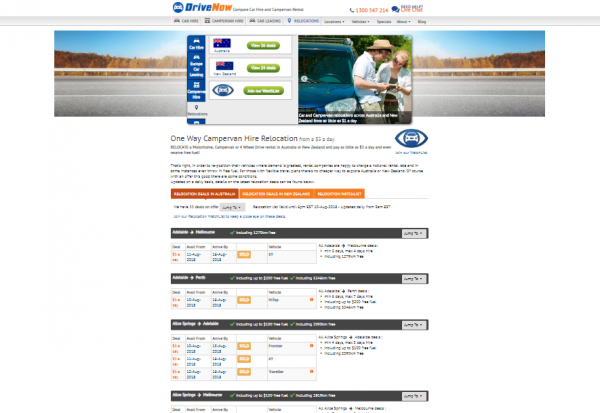Caption: 

A detailed webpage screenshot from "Drive Now," a driving relocation business prominently showcasing their offerings. At the top of the page, the banner displays the company name "Drive Now" along with a contact phone number. Below the banner is a picturesque image of a highway bordered by trees, under a clear sky. 

The central section of the webpage features several clickable links or buttons, likely leading to different services or information. On the right side of the image, there is a car with two individuals standing beside it, seemingly consulting a map or directions. Further down on the right, the same road image reappears.

Beneath this image, there is a notice about "one-way camper van hire relocation," indicating it as a service offered, although the exact price is obscured. The lower section of the page contains detailed information including important trip dates, departure and arrival details, and potentially the routes covered, despite being too small to read clearly in the screenshot. The overall impression is that the business specializes in vehicle rentals and relocation services, possibly offering one-way hires and assistance in moving.